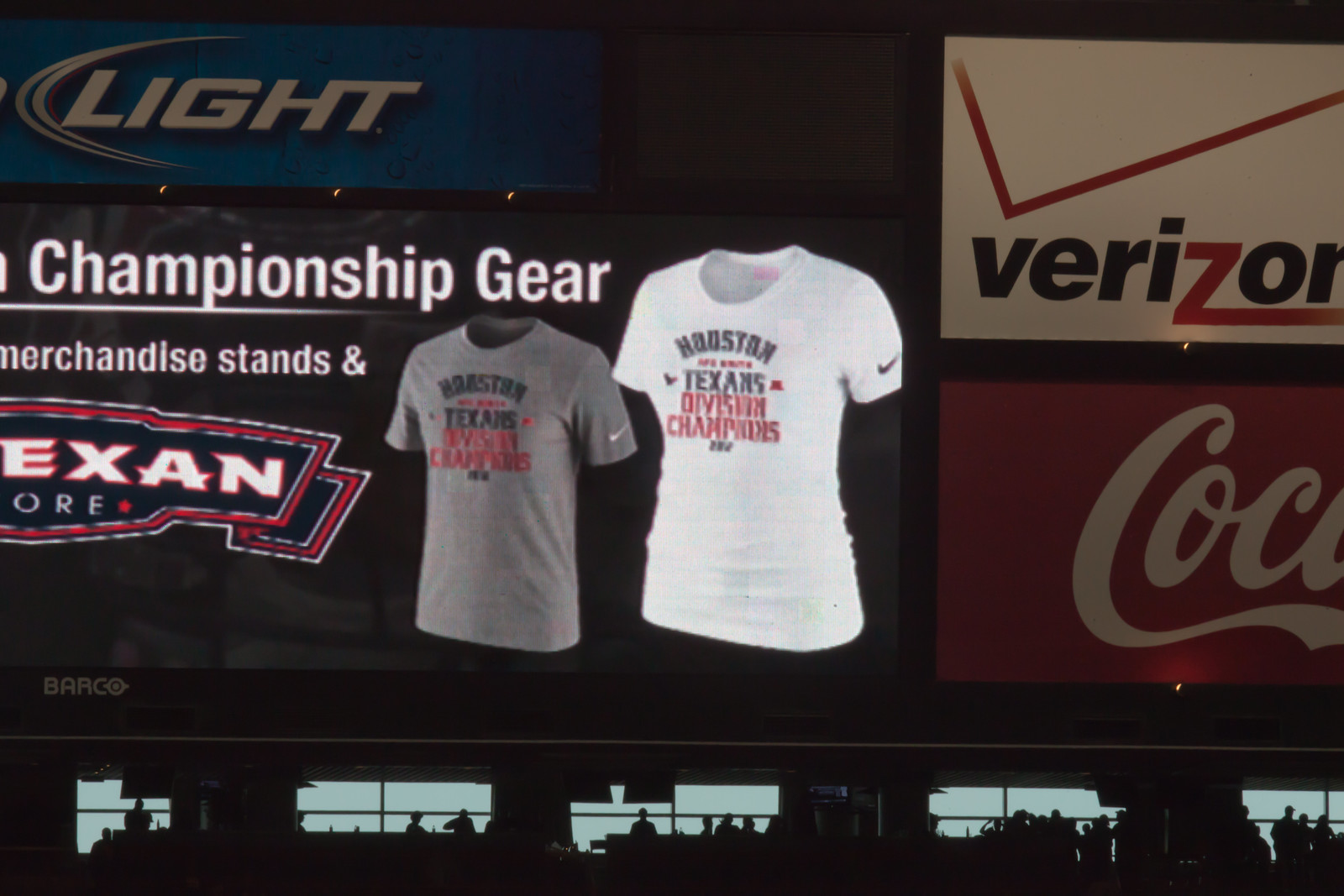The image captures a digital display inside a stadium, showcasing multiple advertisements and merchandise. In the top left corner against a black backdrop is the Bud Light logo, with only the word "Light" visible in large, italicized, all-capital letters and a faint dark blue rectangle. To the left, a crescent shape can be seen. Prominently displayed in underlined bold white font are the words: "Championship Gear, Merchandise Stands," with a partial view of what appears to be "Texan Store." Below this, two Nike T-shirts are advertised—one gray men's shirt and one white women's shirt, both bearing the Houston Texans, Division Champions branding. On the right side of the screen, there are partial logos with a distinct white Verizon logo, where the "Z" is highlighted in red, and beneath it, the beginning of a red Coca-Cola sign. The background shows parts of the stadium, possibly including luxury boxes with spectators.